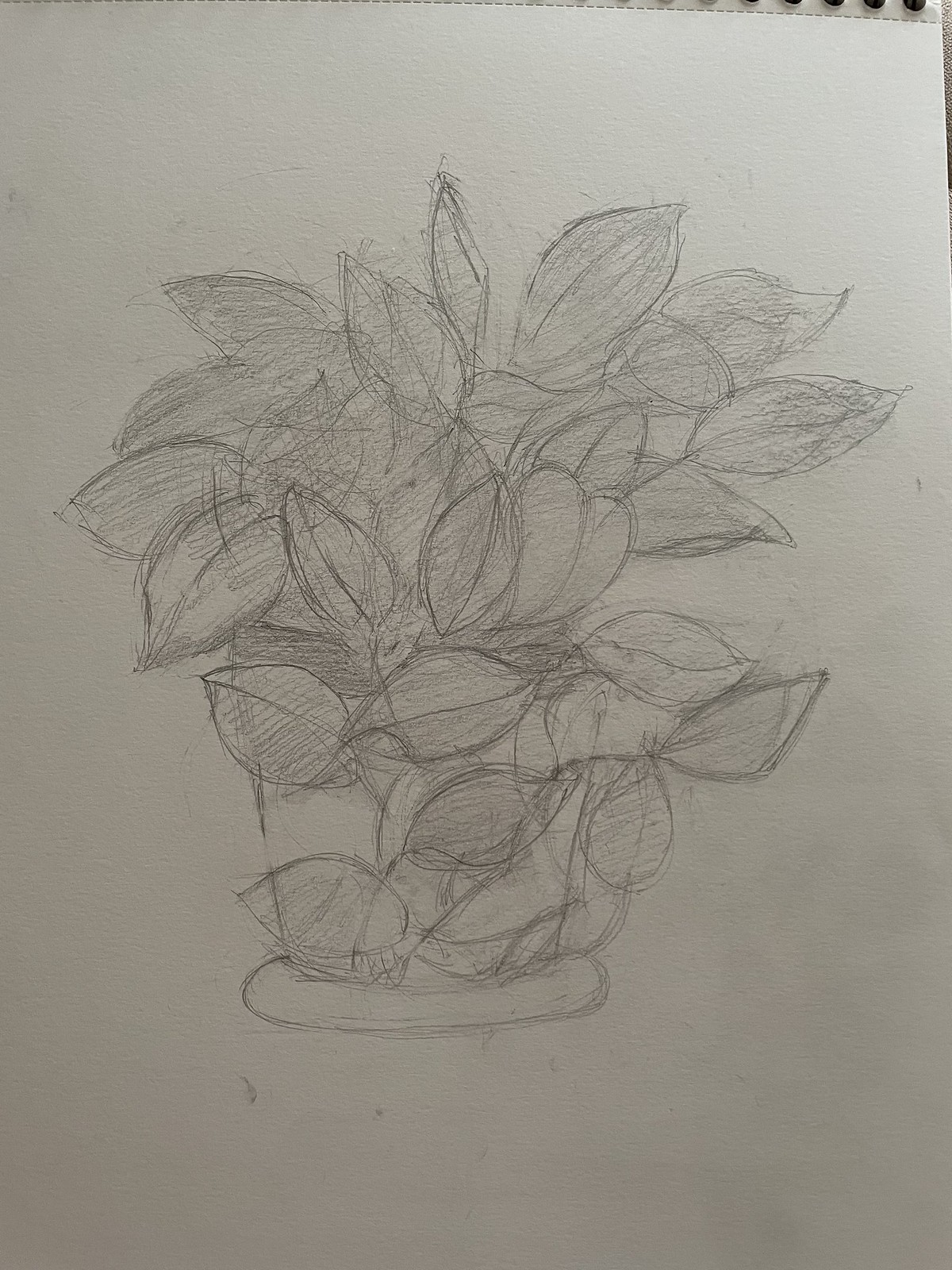This color-capable photograph, presented in portrait format, captures a detailed pencil sketch of a potted plant on what appears to be a high-quality, thicker A4 sheet of paper. The sketch, done predominantly in shades of light gray and black, vividly portrays a simple pot enveloped by numerous large leaves. These leaves cascade around the pot, covering its top and sides, and some extend over and beyond the pot's rim. The base of the pot sits atop what looks like a cushiony cylinder. The sketch employs subtle shading techniques, possibly involving both pencil and charcoal, to give depth and dimension to the otherwise plain composition. Perforated lines visible at the top right hint that the paper could be from a notebook. Despite the detailing in the plant's leaves, which vary in their shading intensity, the image remains focused solely on the pot, the leaves, and the base, with no additional elements or signature present.